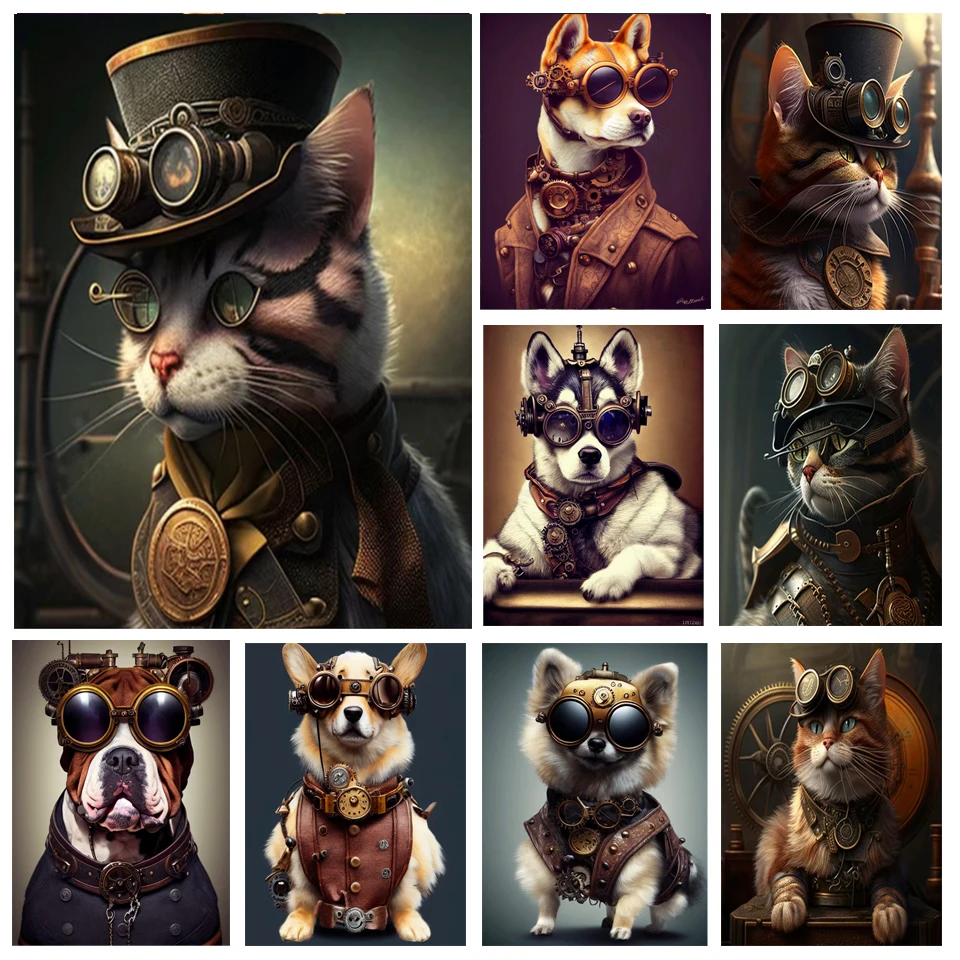The photo is a captivating collage of creatively dressed cats and dogs, exuding a retro yet steampunk aesthetic. The collage is divided into nine sections, with the upper left-hand corner featuring a large, prominent image of a cat that occupies two-thirds of the top portion and half of the left side. This central cat sports aviator glasses, a brown top hat with bronze goggles, a blue coat adorned with buttons, and a large gold pendant. Its face also showcases tiger stripes, all set against a green and yellow background. Surrounding this central image are eight equally sized pictures of various dogs and cats, each donning an array of striking accessories. Among them are a Shiba Inu, a Boston Terrier that resembles a Chihuahua, an orange tabby cat, and another striped tabby cat. These animals are outfitted with steampunk goggles, monocles, leather vests, and leather armor, all emanating a Victorian-era style infused with a steampunk flair. The ensemble of images collectively presents a playful yet sophisticated look, blending elements of vintage and futuristic fashion.